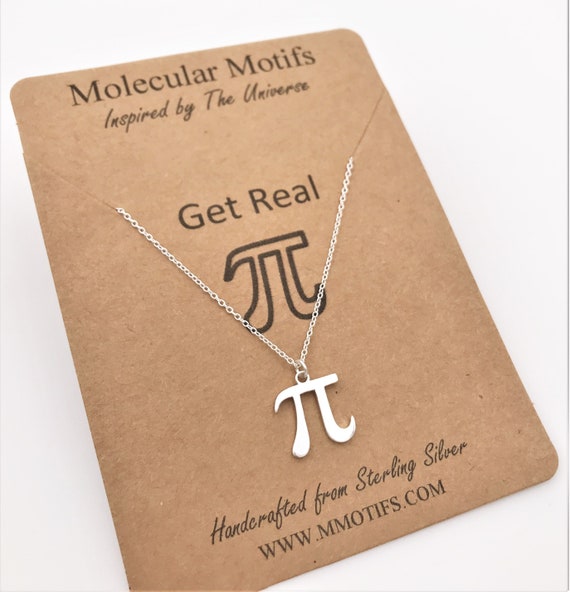The zoomed-in photograph captures a striking necklace displayed on a brown rectangular card. At the top, embossed in darker brown text, it reads "Molecular Motifs Inspired by the Universe." In the center of the card is the phrase "Get Real" alongside a black outline of the Pi (π) symbol. The necklace, which features a silver Pi symbol pendant, is elegantly suspended from a thin silver chain. The bottom of the card states, "Handcrafted from Sterling Silver" along with the website "www.mmotifs.com." The entire arrangement, including the brown card and necklace, is set against a plain white background, giving the impression of an advertisement showcasing the fine details and craftsmanship of the piece.